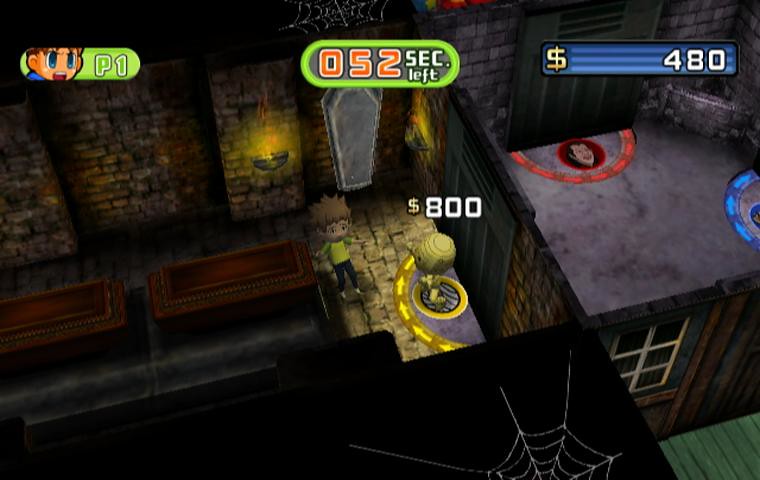The screenshot depicts a retro video game with a low-quality, cartoon animation style. The game is presented from a top-down perspective, showcasing a stone-like castle environment with cobwebs in the upper portion of the image. Centrally, there's a figure of a man with spiky brown hair, dressed in a green shirt and pants, positioned facing a coffin. Above this character, in red font, the timer indicates "52 seconds left."

To the top left, an icon featuring a boy's face with large eyes and an open mouth is labeled "P1," likely indicating Player One. On the top right, a blue bar displays "$480." In the middle of the screen, a yellow, round-headed character with $800 written above it stands in front of the coffin, suggesting an antagonist or valuable target in the game. There are lit torches on the stone walls and adjacent rooms within the castle, one of which features a reddish coffin and another appears to have a wooden wall with a window with blue shutters. Additionally, there's a red, cartoonish vampire-like figure on the cement floor, adding to the eerie atmosphere of the scene.